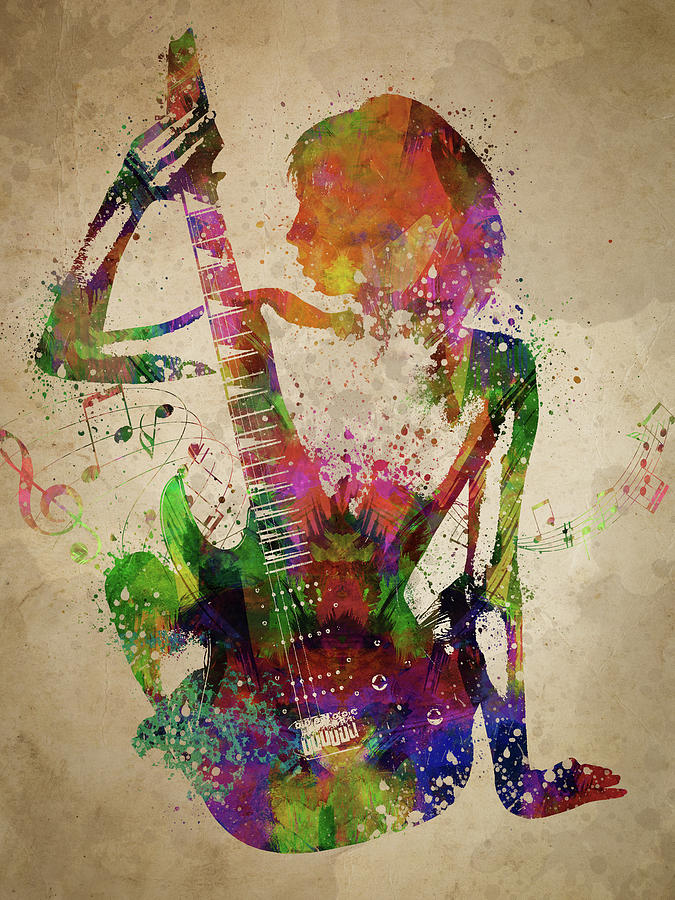This digital art piece features a striking silhouette of a woman with a short bobbed hairstyle, holding an electric guitar. The background is composed of swirling shades of tans and grays, resembling antique, water-stained paper. The woman’s silhouette, rendered in watercolor paint splatters of vibrant colors including greens, pinks, oranges, blues, purples, neon yellow, and turquoise, stands out against the muted backdrop. Her profile faces to the right, and her left hand firmly grips the neck of the guitar, which cascades down alongside her legs. The silhouette of the guitar, like the woman, is textured with splattered watercolor layers. A dynamic wave of musical notes strings across the center of the piece, adding a sense of movement and melody. Scattered paint speckles envelop both the woman and the guitar, enhancing the lively and fluid nature of this digitally crafted artwork.